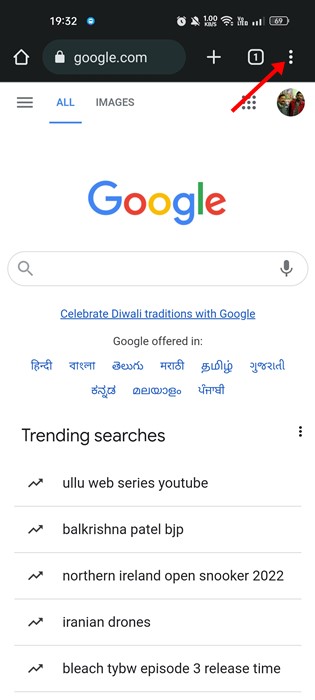**Descriptive Caption:**

The image depicts a screenshot of the Google homepage with a predominantly white background. At the top of the screen is a black rectangular box displaying the year "1952" accompanied by a small blue circle. Below this, there is a horizontal sequence of icons: a battery symbol, a house icon, a padlock, the text "google.com," a plus sign, and a small square with the number "1" inside it. 

A long red arrow points upwards towards a cluster of three vertical dots, likely indicating additional options or a menu. Directly below the black box on the white background, there are three light gray horizontal lines.

Below these elements, highlighted in blue and underlined, is the word "All," followed by "Images." Next to these, there is an icon comprising nine small dots arranged in a grid pattern and a circular icon containing an unspecified image.

The central portion of the page features the colorful Google logo, with letters in blue, red, yellow, and green. Beneath the logo is a search box with the placeholder text "Celebrate DeWalt traditions with Google." Just below the search box, additional text notes that Google is offered in various languages. Further down, a section labeled "Trending Searches" lists five current popular search terms, each accompanied by a small, angled arrow indicating more options. The trending searches displayed are:

1. Ulu, Web Series YouTube
2. Balkrishna Patel BJP
3. Northern Ireland Open Snooker 2022
4. Iranian Drones
5. Bleach Thai BW Episode 3 Release Time